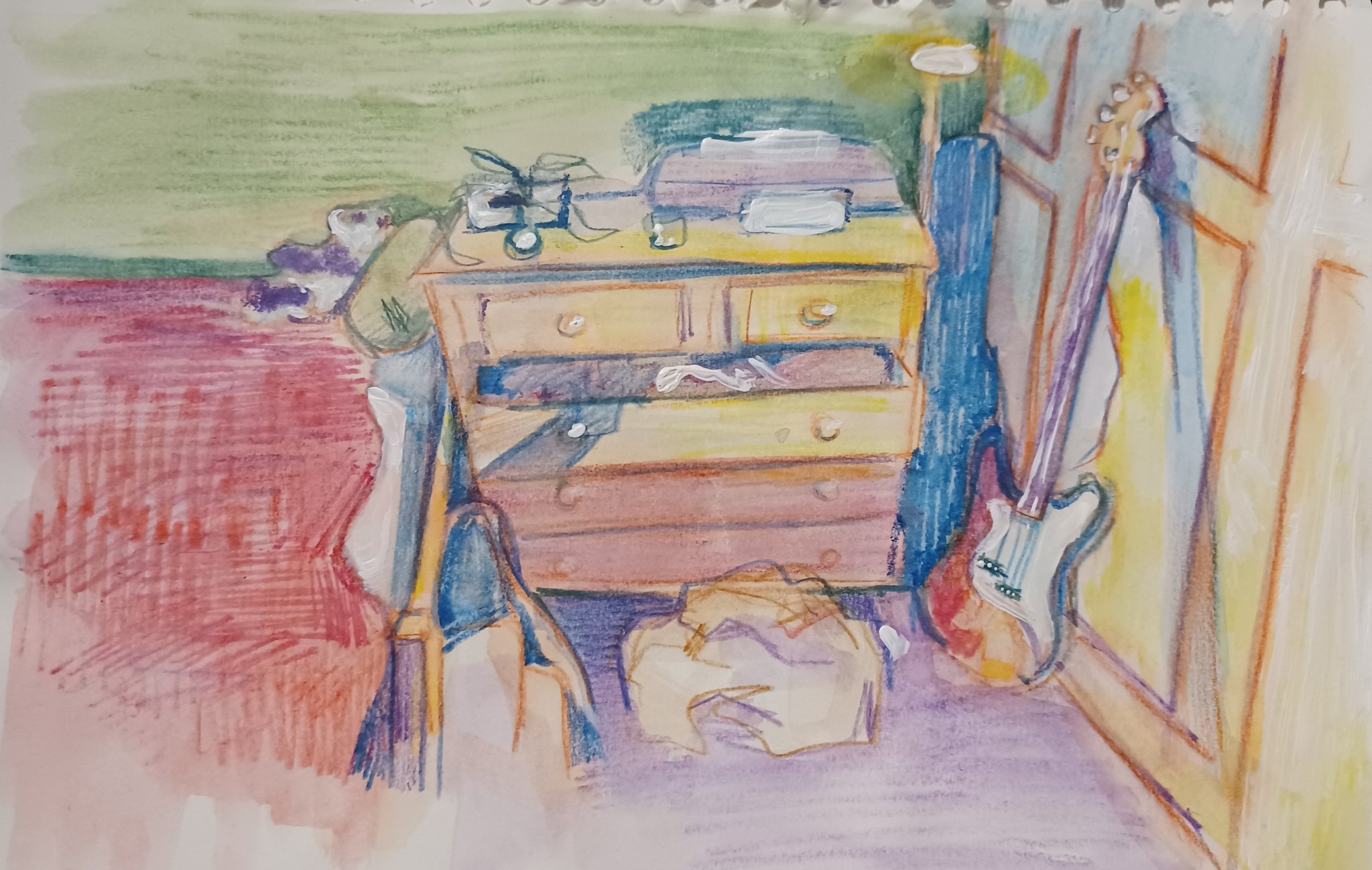This colored pencil drawing depicts a cozy bedroom adorned with vibrant and nuanced details. The room is anchored by a plush purple carpet that adds a touch of warmth. Centered in the space is a white bed with a sturdy brown frame, draped with a red blanket. The backdrop features a striking green wall, while the adjoining white wall to the right is decorated with rectangular art pieces. Leaning gracefully against this white wall is a guitar with a striking two-tone palette of a white and red body and a brown neck, accompanied by a guitar case nestled in the corner. 

To the left, a curious white shape on the floor, resembling a crumpled pile of clothes, adds a lived-in feel. Adjacent to this is a wooden dresser characterized by two small drawers at the top and three larger drawers below. Atop the dresser sits a printer with a sheet of white paper ready for use. Additionally, there is a white square object with a distinct black component emerging from it, possibly a charging station or a small lamp. A slightly open drawer reveals neatly arranged clothes within, adding further realism and depth to this charming scene.